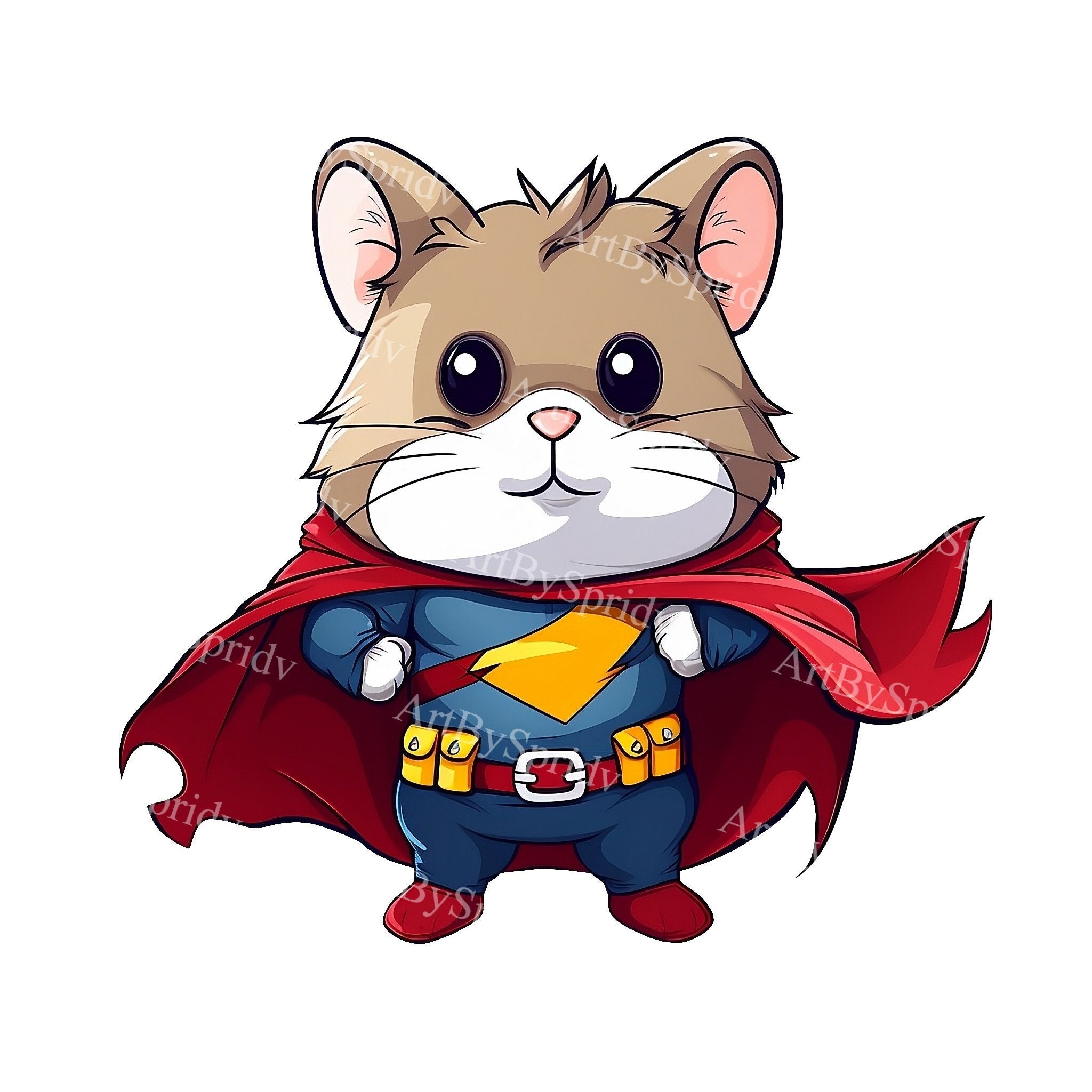This image is a detailed cartoon drawing of a superhero hamster, signed by the artist "Art by Spirid" and marked with noticeable watermarks. The character is a small, brown hamster with black whiskers, a white mouth, and a tan head featuring pink ears and a small pink nose. Its eyes are black with white highlights, giving it a lively expression as it stares straight ahead with a slight smile.

The hamster is dressed in a vibrant superhero outfit, including blue pants, a blue shirt, and white paws. A flowing red cape is securely fastened around its neck and extends behind it, emphasizing its heroic stance. The hamster also wears red shoes and a red belt equipped with yellow pouches for carrying items. A prominent yellow sash with a red and blue ribbon is draped across its chest, adorned with a yellow rectangle that seems unfinished. The background of the image is entirely white, making the colorful character stand out even more.